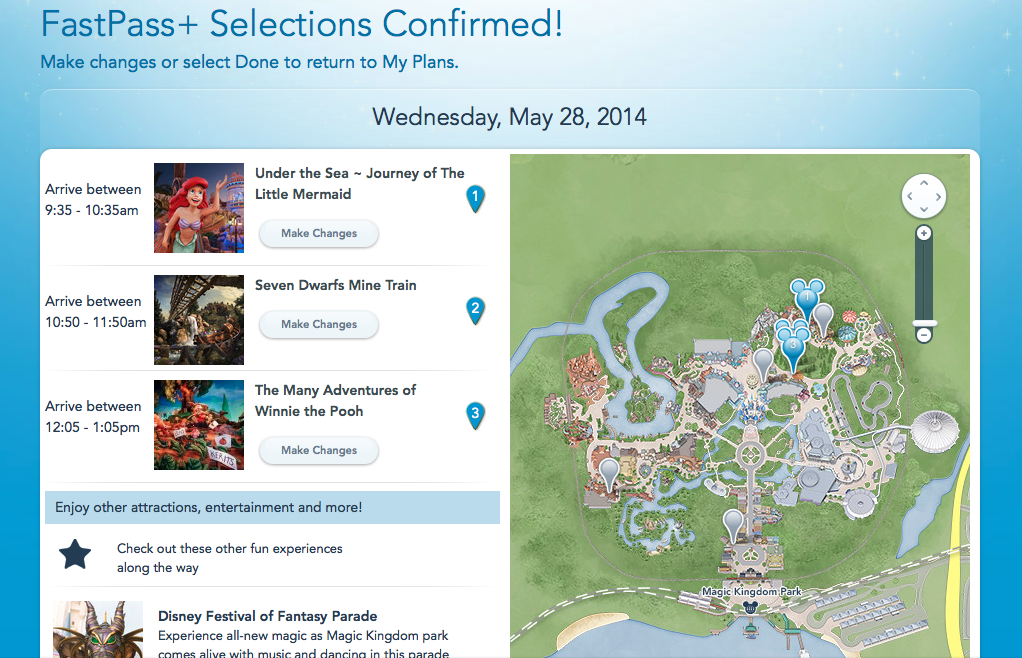The top of the page displays a header stating "FastPass+ Selections Confirmed," accompanied by instructions to either make changes or select "Done" to return to the user's plans. The detailed schedule is as follows for Wednesday, May 28, 2014:

1. **Under the Sea – Journey of the Little Mermaid**: 
    - **Arrival Window**: 9:35 AM to 10:35 AM
    - **Description**: The attraction features a depiction of the undersea world with the Little Mermaid herself.

2. **Seven Dwarfs Mine Train**: 
    - **Arrival Window**: 10:50 AM to 11:50 AM
    - **Description**: Illustrated with an image of a train and the Seven Dwarfs from the classic Disney tale.

3. **The Many Adventures of Winnie the Pooh**:
    - **Arrival Window**: 12:05 PM to 1:05 PM
    - **Description**: This section includes an image of Winnie the Pooh sitting contentedly by a tree.

The page also encourages visitors to "Enjoy other attractions and entertainment and more," highlighting the **Disney Festival of Fantasy Parade**. This parade promises a magical experience, bringing Magic Kingdom Park to life with vibrant music and dancing.

A map of Magic Kingdom is provided, with markers indicating the locations of the featured attractions:
- **Under the Sea – Journey of the Little Mermaid** (Number 1)
- **Seven Dwarfs Mine Train**
- **The Many Adventures of Winnie the Pooh**

The detailed itinerary and additional experiences suggest a well-planned day of enjoyment at the Magic Kingdom.